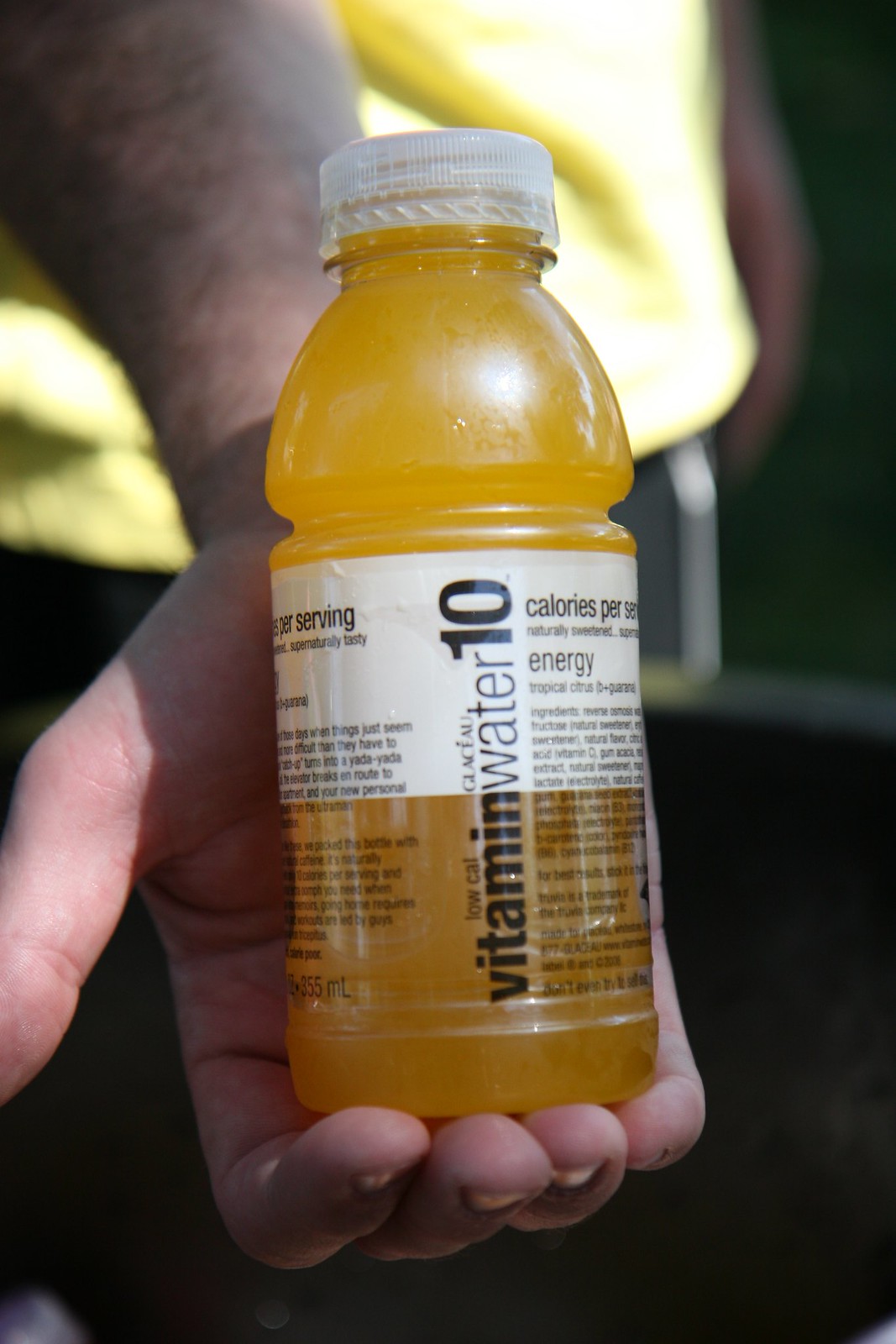The image depicts a clear plastic bottle of Vitamin Water 10, filled with a golden-orange liquid. The bottle features a partly clear label with the top portion being white and the bottom part transparent. Its clear, twist-off cap tops the bottle, which prominently displays the text "Vitamin Water 10," indicating its low-calorie content and energy-boosting properties. A Caucasian hand, with visible hair on the arm, is holding the bottle. The fingers and thumb of the hand wrap around the bottle, with the bottom resting on the fingers.

The background includes a yellow object, which might be part of a tote or an article of clothing, along with a metal stripe and a darker colored area at the bottom of the image. There is some light reflecting off the top right of the bottle, possibly from the sun or a camera flash, and indistinct whitish shapes in the lower-left and upper-right corners of the image. The surroundings and additional elements are vague but add a sense of depth and context to the image.